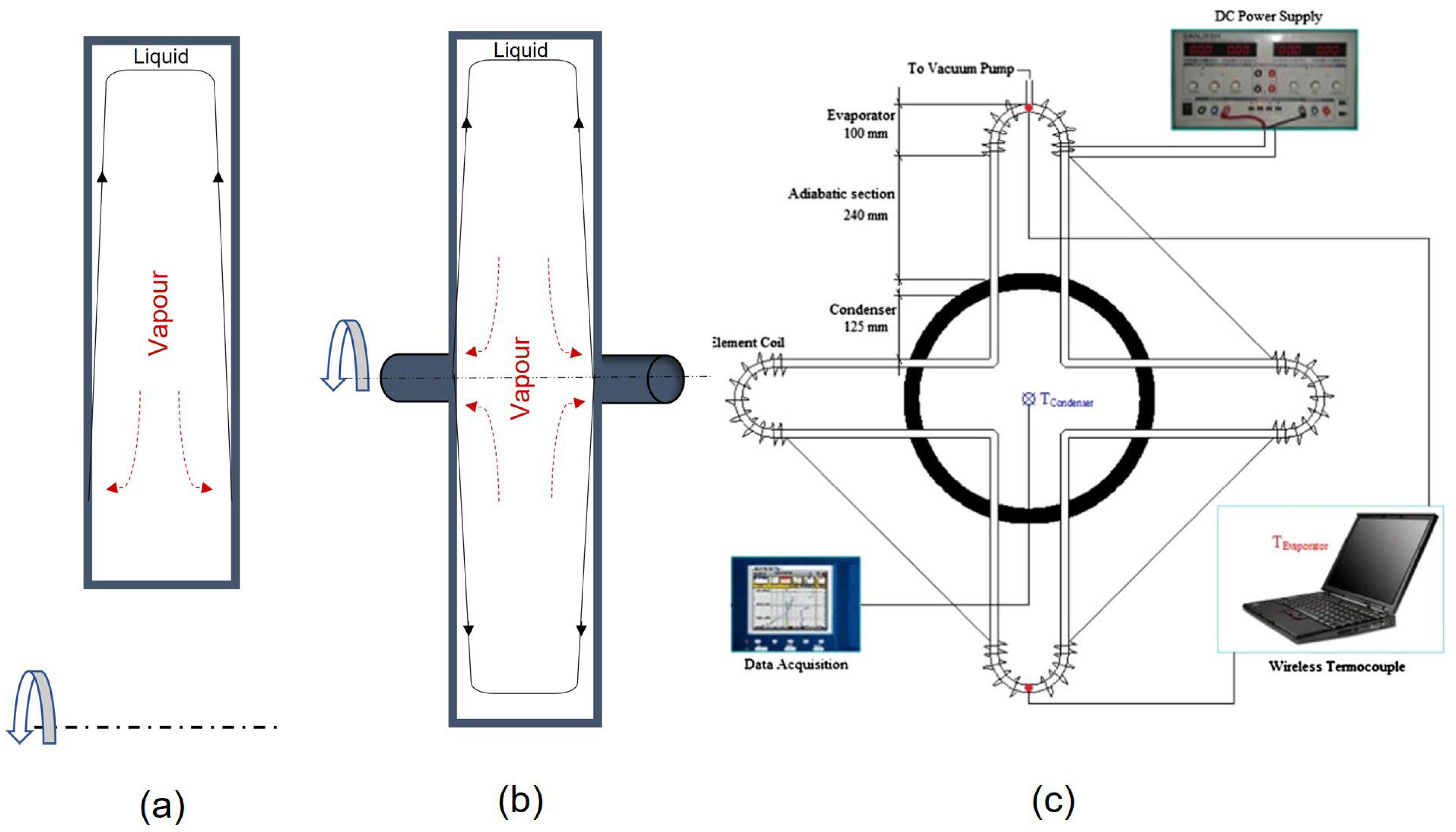The image depicts a detailed schematic, likely from a scientific or technical source, such as a computer screen displaying a diagram from a science book or a research paper. The left side of the diagram prominently features two rectangular boxes labeled as "Item A" and "Item B," both containing the terms "liquid" and "vapor." Moving to the center, there is a large circle with a cross-like structure, connected to various components on the right side. The right side includes several labeled items: a "laptop," "wireless thermocouple," "DC power supply," "data acquisition," an "element coil," an "evaporator," and a connection "to vacuum pump." These elements are interconnected by lines, suggesting an experimental setup possibly related to vapor-liquid interactions. Various knobs, dials, and wires are also depicted, indicating a complex system likely used for data collection and monitoring in a scientific experiment.